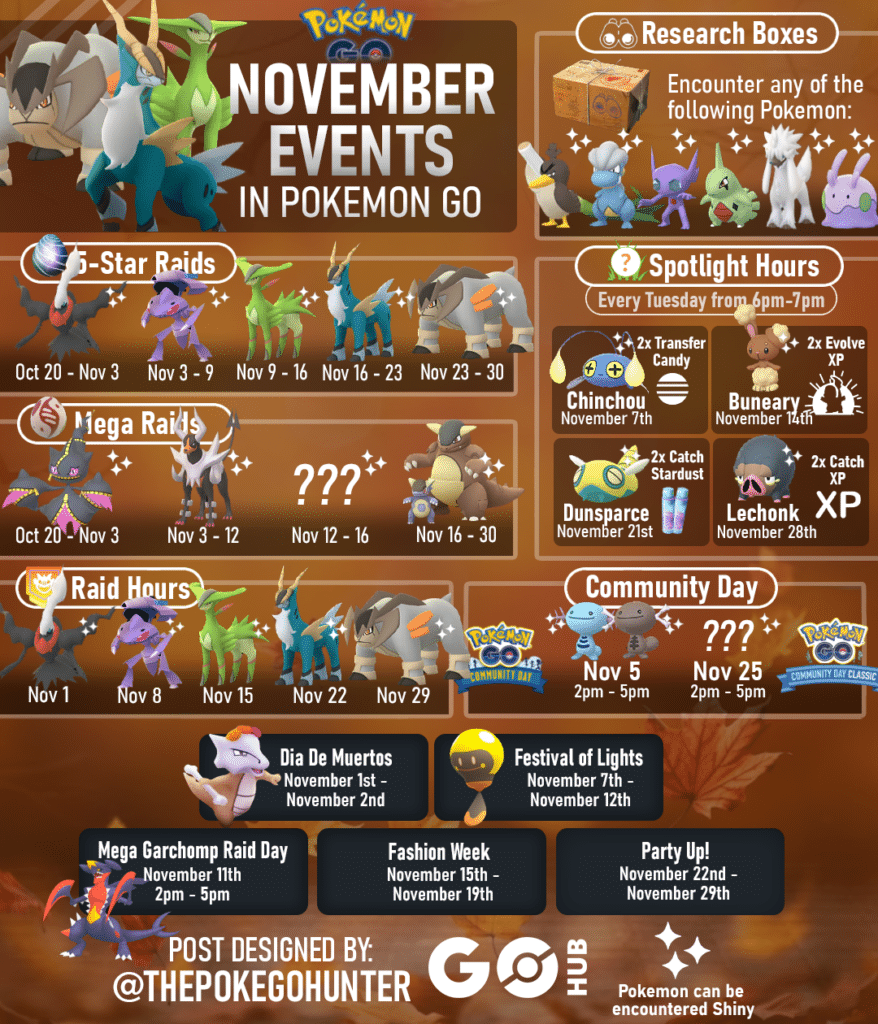This poster for Pokémon GO features an array of exciting events happening throughout November. The prominent "Pokémon GO November Events" headline is written in bold white letters over a brownish background adorned with autumn leaves. Just below, the classic yellow "Pokémon" logo is curved gracefully above the large blue "GO."

To the left, three Pokémon are displayed: one resembling a round silver armadillo on all fours, another with long, pointy antlers, blue limbs, and a white belly, and a third Pokémon with ears extending outwards and a greenish hue. 

The poster details several event dates:
- **Five-Star Raids**: 
  - October 20th to November 3rd
  - November 3rd to 9th (featuring the Pokémon with extended ears)
  - November 9th to 16th (showing another Pokémon)
  - November 16th to 23rd (blue-limbed, antlered Pokémon)
  - November 23rd to 30th (round silver armadillo-like Pokémon)

- **Mega Raids**: Four different characters are listed, with one shrouded in mystery, indicated by a question mark.

To the top right, the poster highlights research boxes, inviting players to "encounter any of the following Pokémon." The right section also mentions "Raid Hours" and "Spotlight Hours" happening every Tuesday from 6 to 7 PM, offering rewards like XP or other bonuses.

Additionally, it celebrates "Community Day" and other partner events including:
- Fashion Week
- Party Up
- Mega Gorcha Parade
- Fossil Lights
- Dia de Maracas

At the bottom, it states: "Poster designed by the Pokémon GO Hunter," alongside the note that Pokémon may be encountered in their Shiny forms, signified by sparkling star icons.

This visually appealing and information-packed poster ensures Pokémon GO players are well-informed about the myriad events and special Pokémon appearances throughout November.